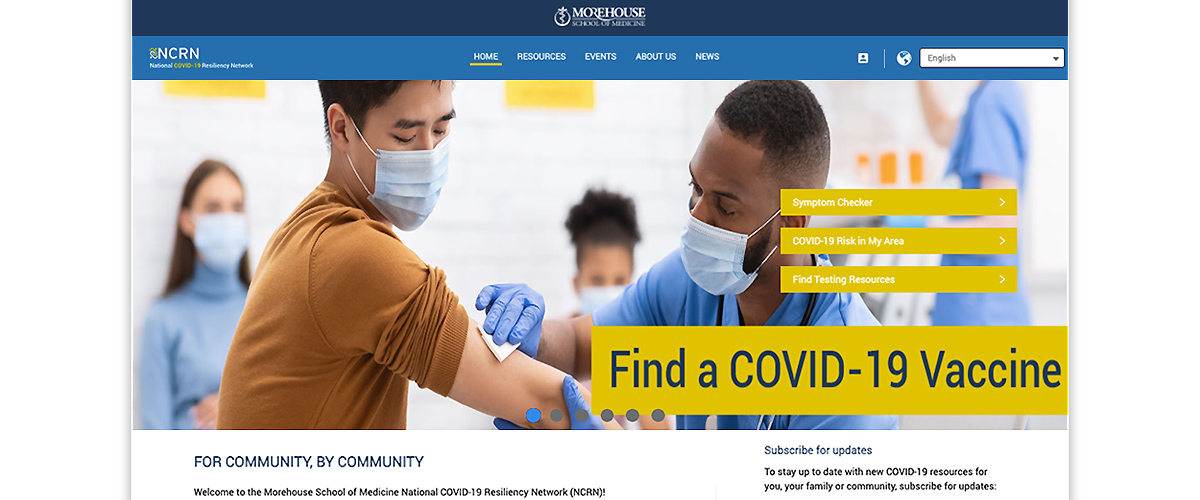This image is a snapshot of the Morehouse School of Medicine website, prominently featuring their National COVID-19 Resiliency Network (NCRN). At the top of the page, menu options are displayed including "Home," "Resources," "Events," "About Us," and "News," with a language selection option to the right. The main focus of the site is to assist users in finding a COVID-19 vaccine, offering a symptom checker tool, local COVID-19 risk assessment, and testing resources.

The image itself shows a busy clinic scene where everyone is wearing face masks. In the foreground, two gentlemen are visible, with one of them receiving a vaccine shot. Behind them are three individuals, two women and another person whose head is out of frame. Below the image, a welcoming message reads, "For Community By Community - Welcome to the Morehouse School of Medicine National COVID-19 Resiliency Program." The website also includes an option for visitors to subscribe for updates on COVID-19 related information and resources.